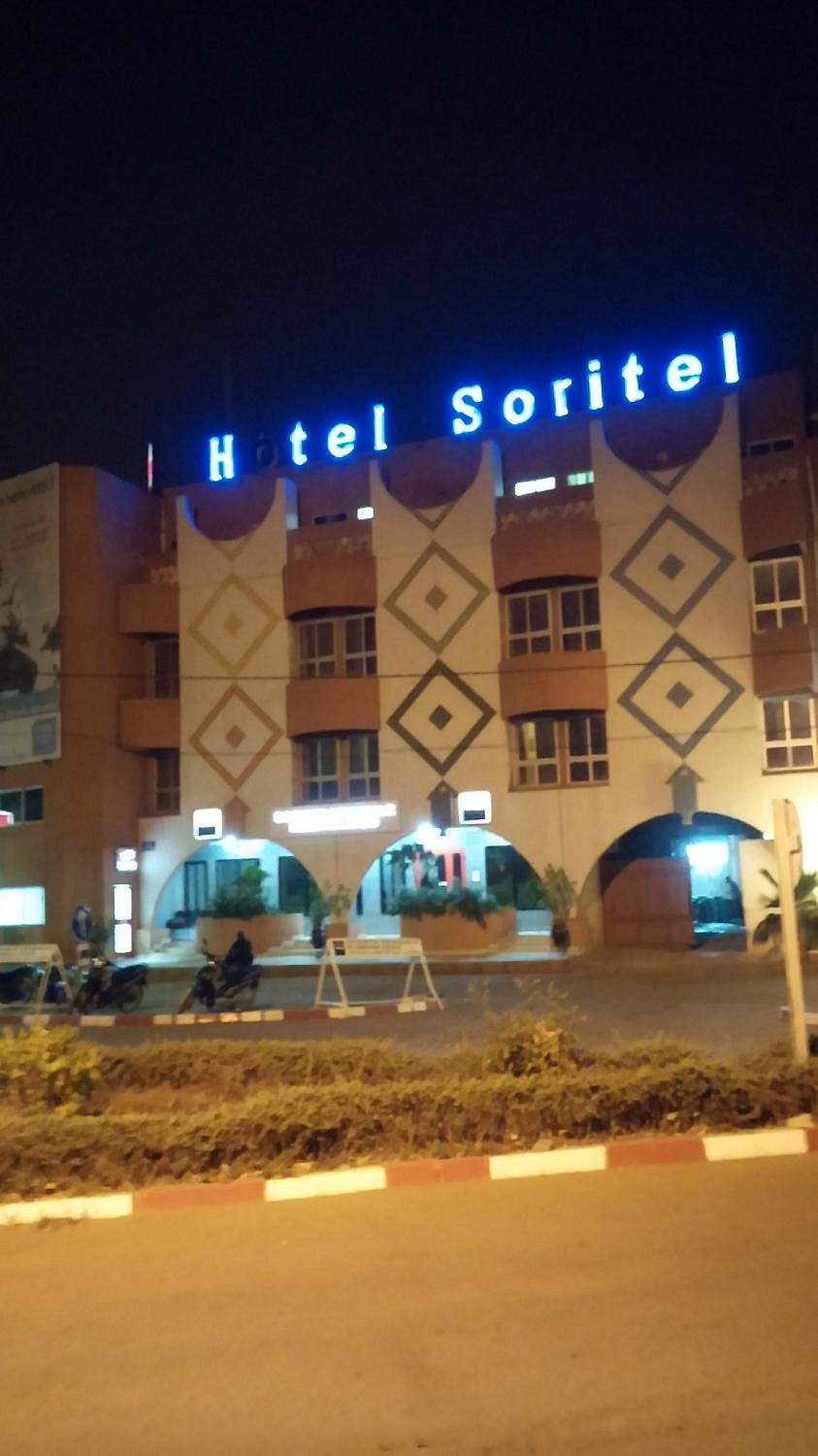This photograph, taken in portrait orientation at night, captures the front facade of Hotel Sorretto, prominently illuminated but for the unlit 'O' in 'Hotel,' making the sign read "H tel Sorretto." The hotel building spans 3 to 4 stories, with architectural elements such as three large pillars adorned with a retro diamond design stretching from the top. Below these pillars are three archways that likely lead to the lobby area. The lower floor is bathed in light, casting an inviting glow. The structure features an off-white and orange color scheme, contributing to its nostalgic charm. The scene is devoid of people and cars, enhancing the emptiness of the street or parking lot, though a few motorcycles and small shrubs can be seen in front of the hotel. The dark night sky provides a stark contrast to the illuminated facade, heightening the visual focus on the hotel.